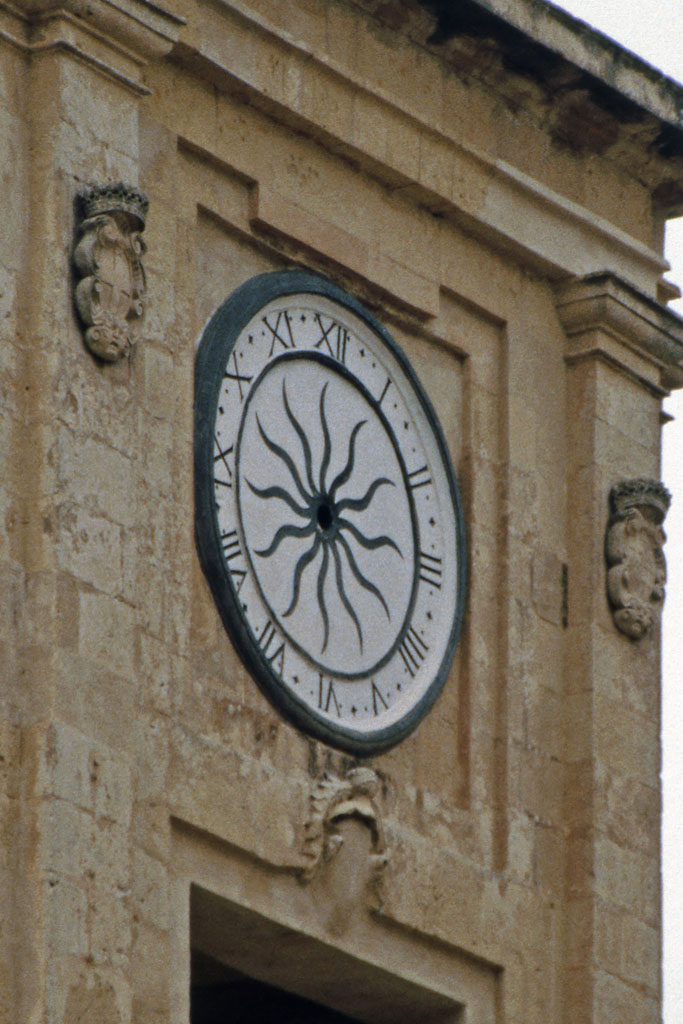This image captures the front facade of the ancient stone building, believed to be the Victoria Citadel in Gozo Island, Malta. The photograph highlights a prominent, old-fashioned clock mounted high above a grand doorway. The stone wall, weathered and aged, has a yellowish-brown hue, evoking a sense of historical grandeur spanning hundreds of years. The clock features a stark white face, encircled by a thick black border and adorned with Roman numerals. A distinctive black sun-like design occupies the center, with a small hole indicating the absence of clock hands. Surrounding the doorway are intricately engraved pillars, each featuring stylized engravings, possibly of goat faces, adding to the ancient aesthetic. Flanking these pillars are what appear to be light fixtures or holders, and beneath the clock lies a small statue, further contributing to the building's elaborate detail and historical significance.